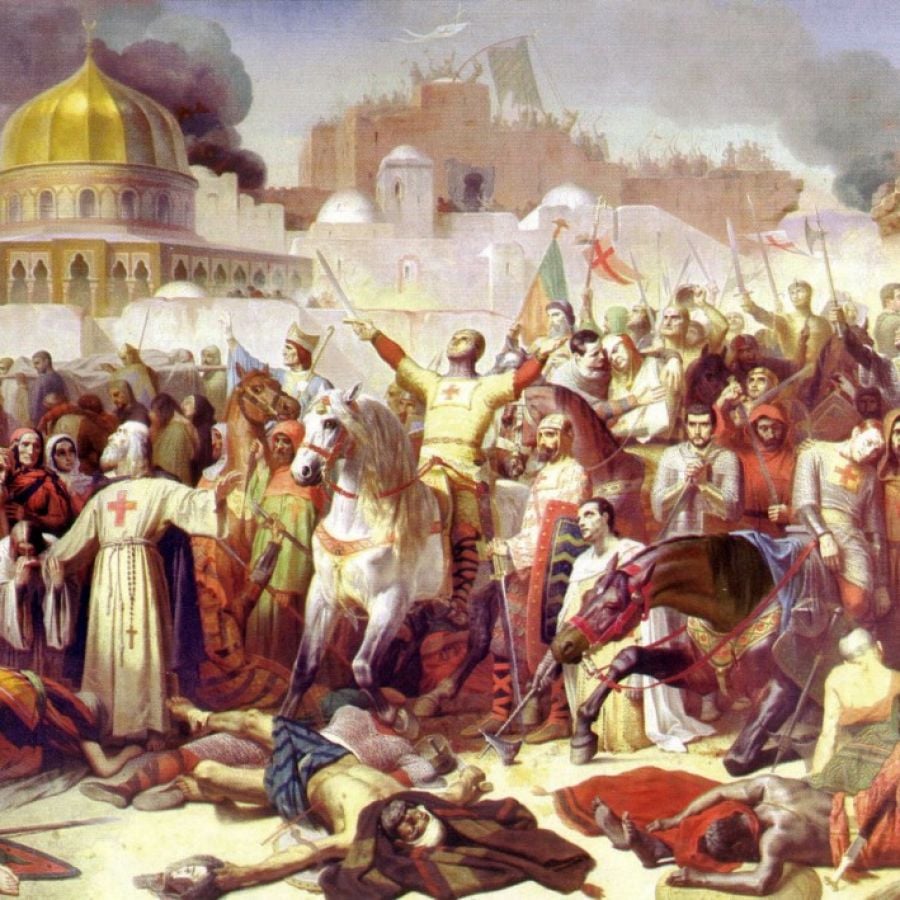The painting depicts a dramatic wartime scene reminiscent of a crusade, likely portraying events from the Renaissance era but with medieval crusade themes. 

In the foreground, a grim tableau of fallen soldiers lies scattered across the terrain, suggestive of a recent violent clash. Among them, mounted knights in white robes adorned with red crosses, emblematic of the Knights Templar, dominate the scene. One notable figure on a white horse raises his sword skyward, his posture exuding a sense of triumph or divine connection. Another Templar, identifiable by his white robe and prominent red cross, stands solemnly over a slain adversary, a cross-tipped chain hanging from his belt. 

The midground is equally chaotic, featuring horses collapsing, either wounded or overcome by the fray, their riders gripping swords raised defiantly in the air. To the left, a large ship is detailed, with a captured flag fluttering above, indicating a significant conquest. Another ship, engulfed in flames, adds to the painting's turbulent atmosphere.

In the background, castle-like structures and a walled city hint at a besieged stronghold, possibly Constantinople, with a distinct golden dome rising above the smoky skyline, further intensifying the scene's historical and cultural resonance. The overall color palette of whites, reds, blues, and yellows enhances the vivid portrayal of this ancient battleground, capturing the essence of a legendary crusade.